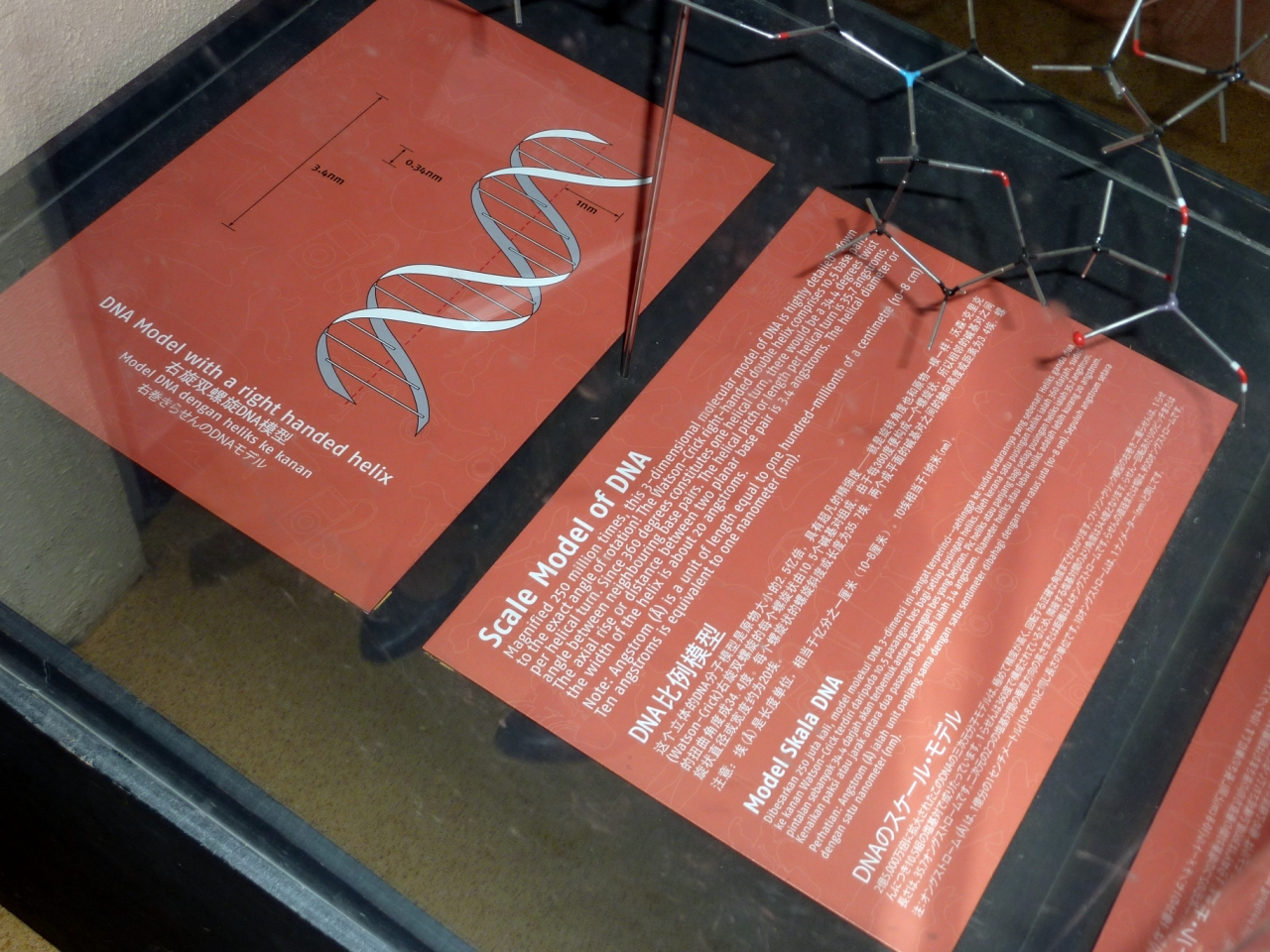The photograph features an intricate model display, likely part of an indoor exhibit in a science museum. Centered on a sleek glass table, the exhibit showcases a sophisticated three-dimensional DNA model composed of silver wires intricately assembled with blue, red, and black connectors, forming hexagonal shapes. The model is supported by a bronze rod emerging from the base of the table. Accompanying the model are red informational placards with prominent white text. The left placard reads "DNA model with a right-handed helix," displayed above an illustration of the helix and accompanied by Asian characters, presumably translations in Chinese and Japanese. The right placard provides a detailed description of the scale model, indicating it is magnified 250 times, along with additional technical details about the molecular structure and rotational angles. This elaborate display provides an educational insight into the structural complexities of DNA.